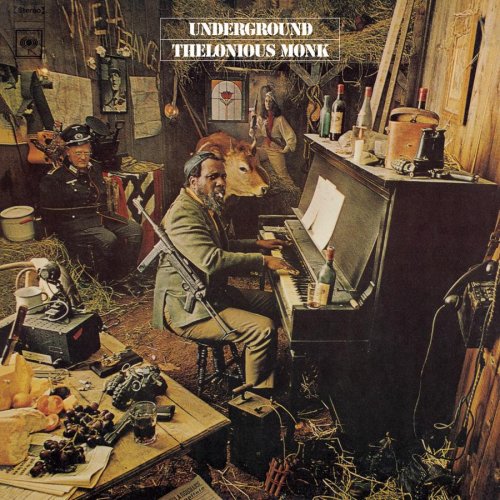The album cover for Thelonious Monk's "Underground" presents a provocative and detailed setting that captures the viewer's attention. In this striking image, jazz legend Thelonious Monk stands resolutely in front of a vintage piano with a cigarette dangling from his mouth, exuding an air of defiance. Slung across his back is an AK-47, further emphasizing the rebellious, wartime mood of the scene. The room around him is both chaotic and meticulously staged, featuring a tied-up SS soldier seated next to a prominently displayed swastika, signaling a clear anti-fascist message. A plunger device for setting off dynamite adds to the palpable tension and intrigue. The space is cluttered with various items that lend it an authentic, underground resistance atmosphere. This cover art not only visually captivates but also stirs curiosity about the album's content and the bold statement it makes.